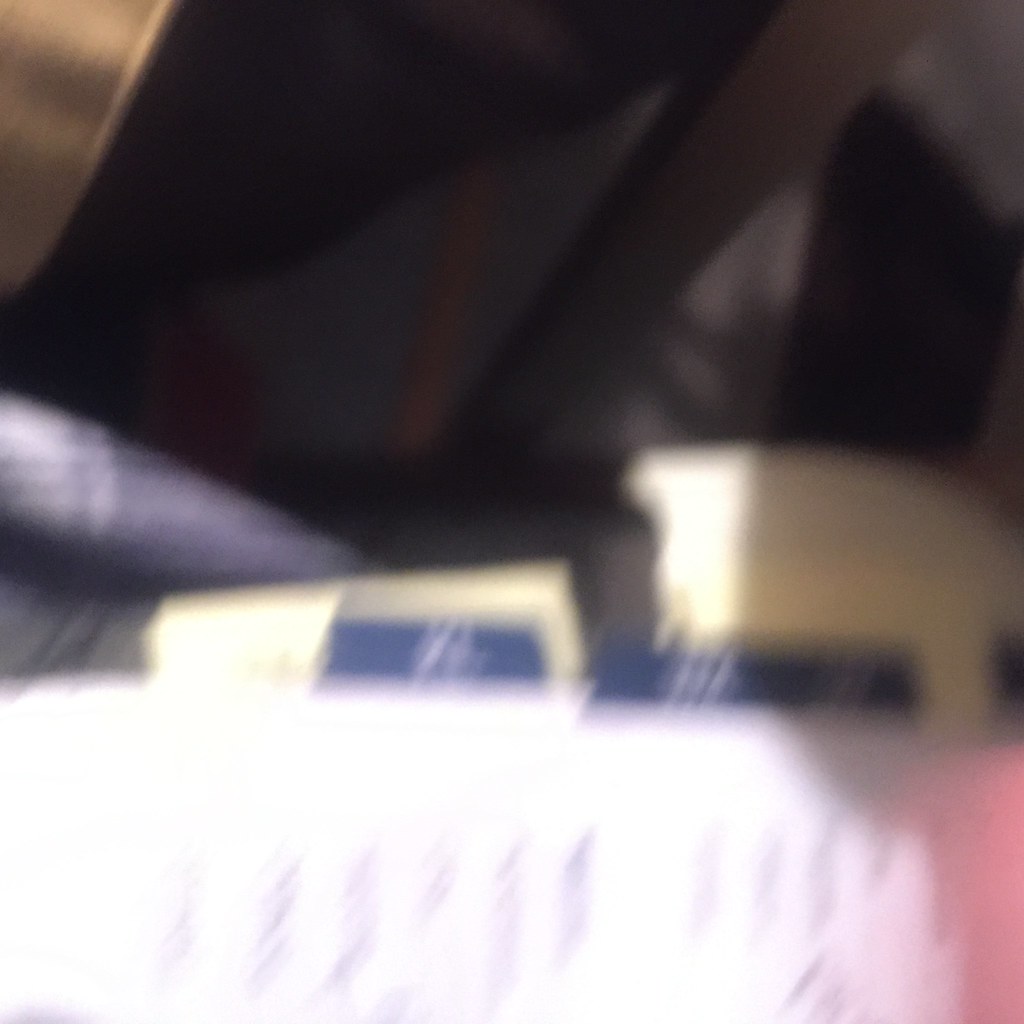The image is extremely blurry and out of focus, making it difficult to discern details. At the bottom of the horizontally oriented photo, there's a piece of white paper featuring some indistinct cursive writing in black. The photo also contains small dark blue labels with blue writing on the side. To the right, there's a piece of scotched cloth with blue and white colors. The background seems to have a black cloth or table with a black pole in the center. There are shadows that could be mistaken for a foot in a black sock, but they are likely just shadows. The overall setting is unclear, but it might be somewhere with close seating arrangements, such as a car, airplane, or waiting room, given the possible presence of a leg next to the paper. There's also mention of other indistinct items which could be a duffel bag or another person. The scene includes a mix of colors like black, white, blue, pink, and tan.